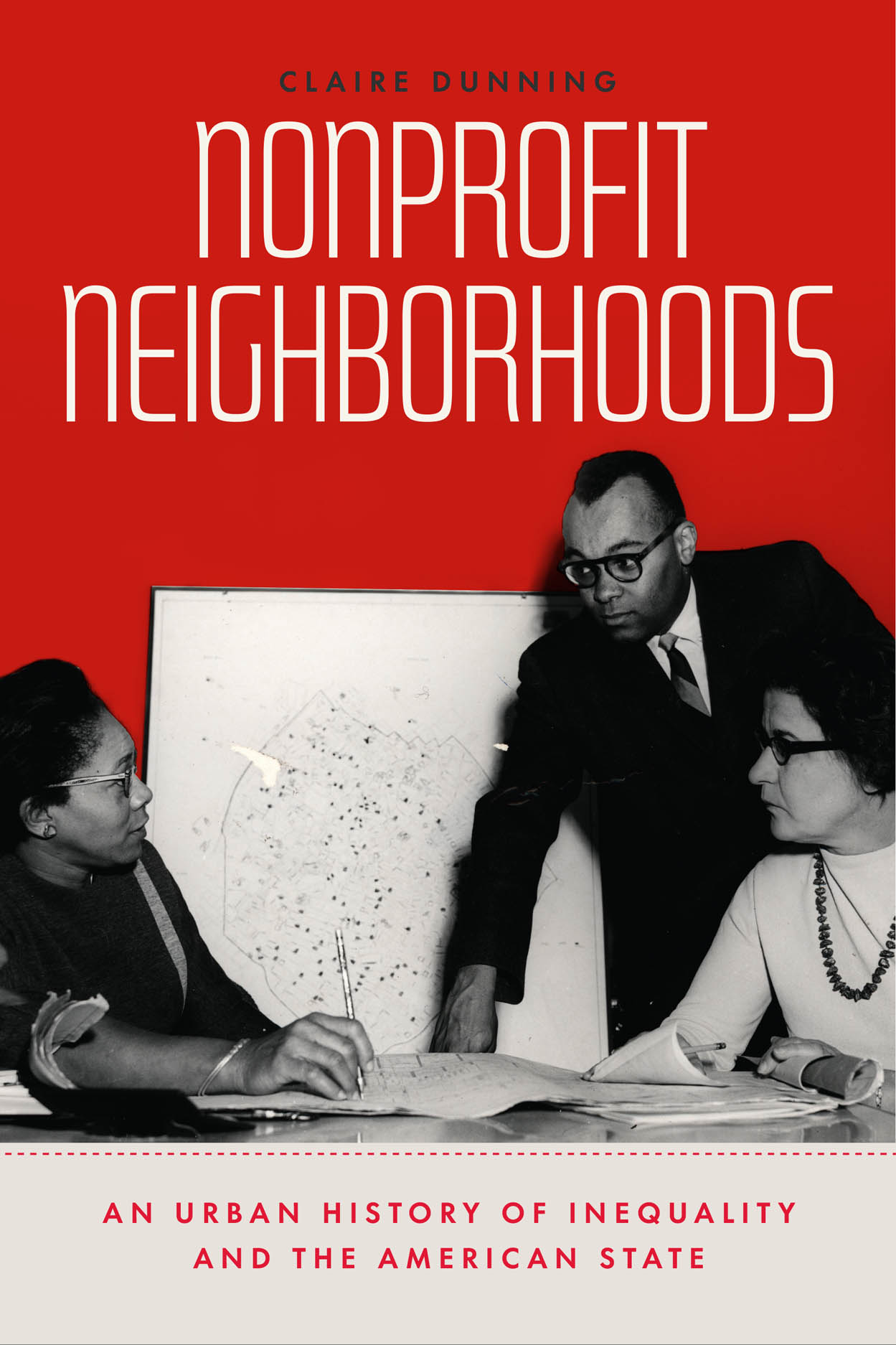The cover of the book features a striking red background with a gray banner at the bottom separated by a dotted red line. At the top, in clear black text, is the author’s name, "Claire Dunning." Below that, in larger white text, reads the title, "Nonprofit Neighborhoods." The gray banner at the bottom contains red text that states, "An Urban History of Inequality and the American State."

Central to the cover image are three people, depicted in black and white, engaged in what appears to be an important discussion or a signing. On the left, a Black woman in a black dress holds a pen in her right hand. To the right, a Black man in a suit and glasses stands over a table with papers scattered on it. Beside him, a white woman also wearing glasses and a necklace sits down, contributing to the conversation. Behind them, a dry erase board displays a map with dots and lines. The image captures a moment of interaction and analysis, underscoring the themes of community and social structures conveyed in the book.